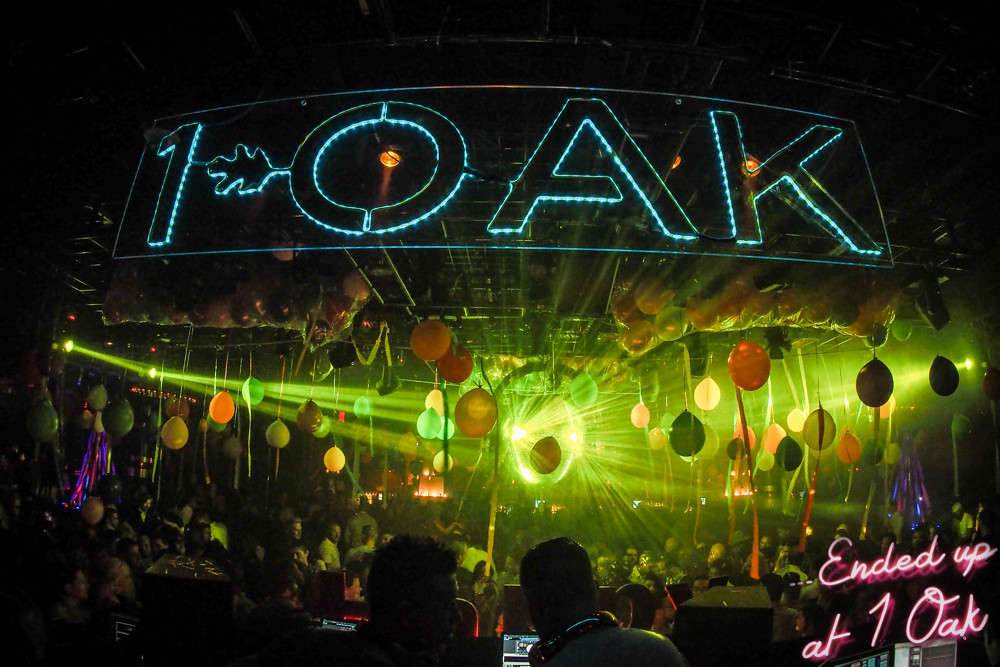This detailed photograph taken from behind the DJ booth captures the vibrant atmosphere inside a club, One Oak. In the foreground, the back of two DJs is visible, one wearing headphones, as they manipulate their musical equipment. Beyond them, a lively crowd fills the dance floor, with some people dancing while others are standing and watching the performance on stage. The ceiling is adorned with colorful balloons, predominantly orange and white, some hanging freely and others encased, ready to drop. Overlooking the scene is an illuminated sign reading "One Oak," created with light blue-colored lights and featuring an oak leaf connecting the "O" and the "One." The entire room is bathed in dynamic green laser lights, enhancing the festive ambiance. In the bottom right corner, edited text in pink cursive reads, "Ended up at One Oak."